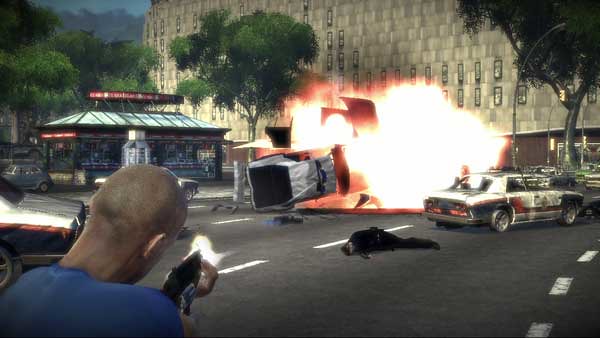The image is a landscape screenshot of a somewhat low-quality video game, characterized by pixelated graphics, particularly noticeable in the green foliage of the trees in the background. In the bottom left corner, the back and shoulders of a bald character wearing a blue shirt are visible as he crudely holds an AK-47-style machine gun, with a bright yellow muzzle blast emanating from it. In the right-center of the frame, a large explosion with yellow and orange edges dominates the scene, sending car parts flying. The explosion seems to involve a blue and white police vehicle, identified by light bars on its roof, which is flipped on its side. In the foreground, the street features white dotted lines and the body of a person dressed in black lying motionless, suggesting police affiliation. To the left of the explosion, another car and a partially visible figure add to the chaotic scene, while the right side reveals another police car amidst the flames. The backdrop includes a large brown building with multiple small windows, vibrant trees, and a structure resembling a kiosk that could potentially be a subway entrance or market stall.